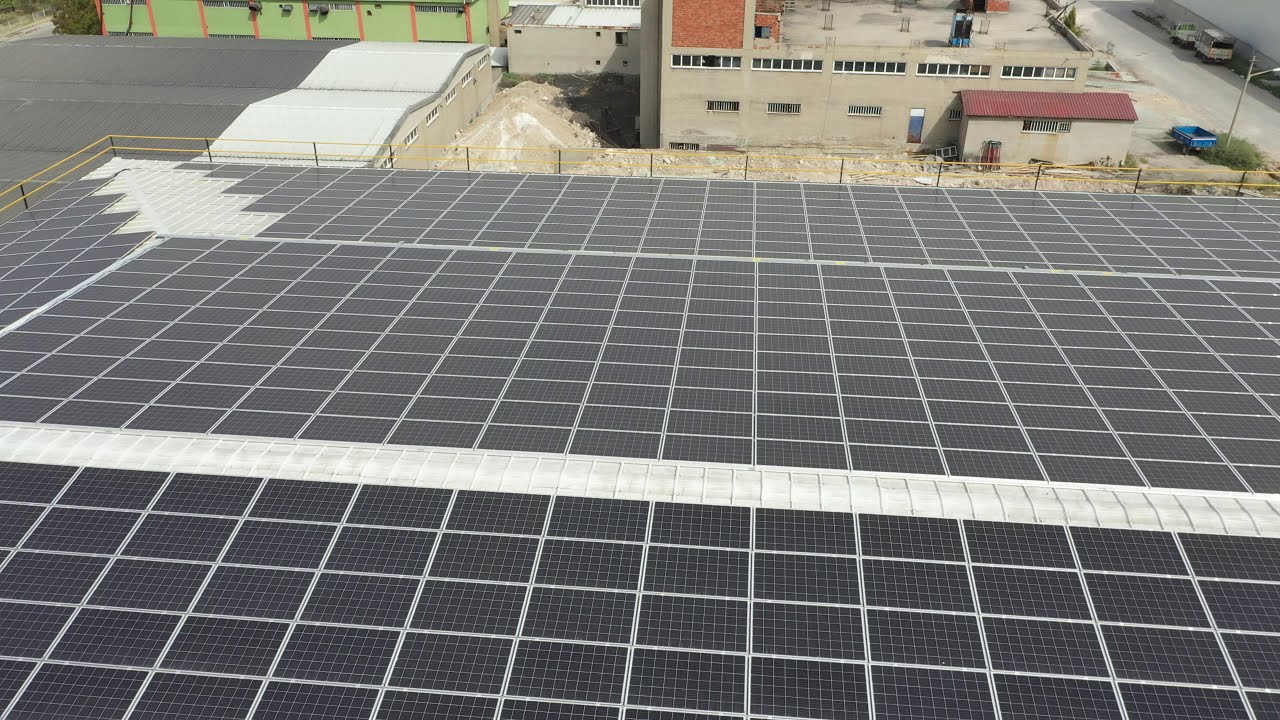The image appears to have been taken from a rooftop, offering a high vantage point over a landscape that includes various buildings, vehicles, and vegetation. Dominating the foreground is a large expanse of slanted solar panels arranged in a grid pattern of black squares outlined in white. Surrounding the solar panel area, which could also be mistaken for black and white bricks or tiles, are yellow poles supported by black poles, forming a barrier on the left side and bottom of the image.

In the upper portion of the image, there are several parked cars in white, gray, and green colors, situated in front of a series of buildings. The central building features a mix of tan and red bricks, complemented by a red rooftop. Adjacent to this building is another structure with similar grayish tones, and to the left, a distinct green building with orange squares and a gray-white roof. Scattered between these buildings are patches of light brown and white dirt, adding to the outdoor setting.

Adding a splash of color, there is a blue wheelbarrow-type trailer near a streetlight and some bushes on the right side. The top left section of the image includes various shades of green trees and bushes. The scene includes no text, and it is difficult to determine the exact purpose of this location, though it could potentially be a school or a similar institution.